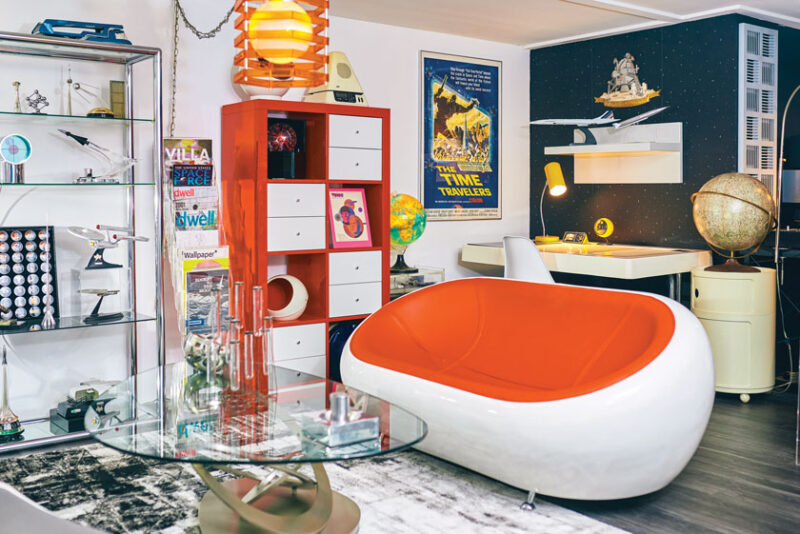The photograph depicts a vibrant, meticulously organized collector's space-age office or a child's themed bedroom, captured indoors under artificial lighting. The overall ambiance is modern with a distinct nostalgic nod to 60s and 70s decor, emphasized by the mix of white and blue walls with white trim. Dominating the central right area, there's a detailed globe on a white stand. 

Towards the left, a sleek white desk and chair are highlighted by a vintage yellow desk lamp. Above this setup is a shelf supporting a detailed model of a jet airplane and other rocket ship models. Ascending slightly, a prominent movie poster for "The Time Travelers" occupies the upper center part of the wall.

The center of the image features another globe, accompanied by a red cabinet fitted with white drawers and assorted collectibles. This area flows into a glass shelf adorned with a myriad of miniature Star Trek ships, other plane models, and various space memorabilia. 

A striking white and orange, pod-like couch with curved edges and a recessed cushion is positioned in front of an oval glass table. The table, which carries an air of futuristic elegance, holds several vials akin to those used in "Star Trek" episodes. 

Accompanying this is a metal and glass display case filled with Star Trek space vessels, rockets, and a variety of space-themed models. There's also a mod bookcase marked by its distinctive ovals and a striking lamp, giving off a 70s vibe, situated above it. Not to be missed is a unique vertical cylinder cabinet with sliding doors, reinforcing the room's eclectic yet cohesive aesthetic.